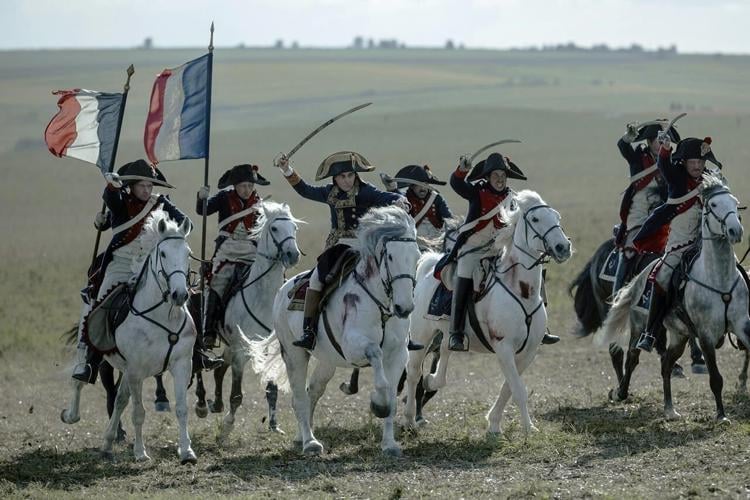In the foreground of a vast, empty grassland, seven French soldiers from the Napoleonic era charge forward on pure white horses. The men, serious and determined, are dressed in elaborate, identifiable uniforms featuring distinctive blue coats, white sashes, and the iconic bicorne hats with elaborate designs. Two soldiers on the far left hold vertical red, white, and blue French flags, while several others brandish curved swords high in their right hands, ready for battle. The central figure's hat is adorned with gold, potentially denoting a higher rank or even Napoleon himself. The horses gallop synchronously from left to right, with no obstructions in the background, creating an evocative and dramatic scene reminiscent of a pivotal moment from history.